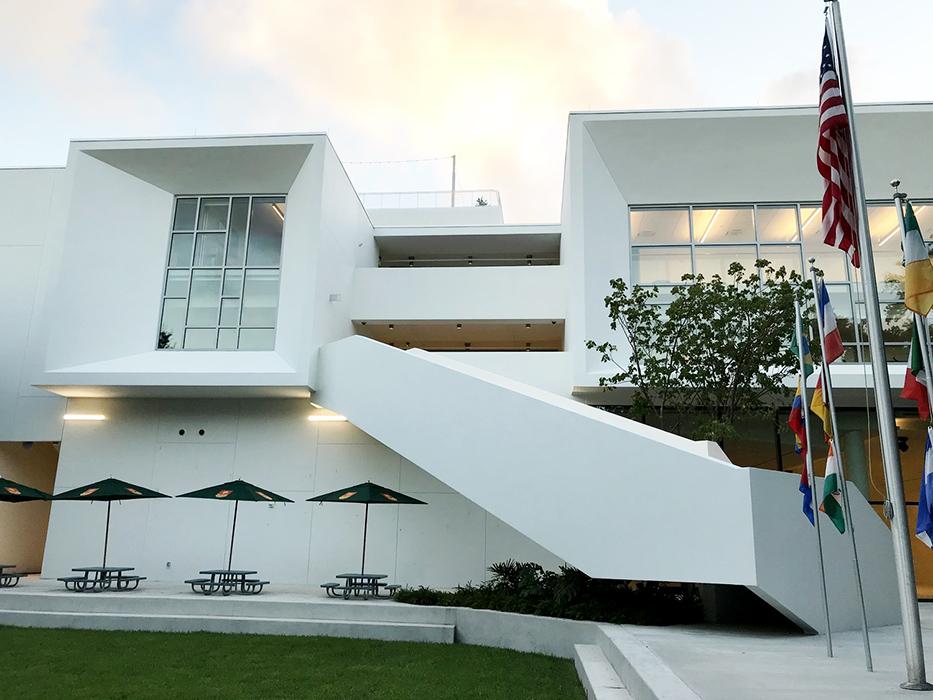The photograph depicts a large, modern white building featuring a sleek and polished exterior, possibly made of smooth stone or cement. The building's architecture is characterized by its box-like, artistic design with windows that protrude outward, creating a dynamic façade. It stands at least two or three stories tall, with prominent large glass windows on both the left and right sides. The left window is part of a square-shaped box, while the right window is part of a rectangular-shaped box.

In front of the building, on the left side, there are four metal picnic tables with black umbrellas, three fully visible and one partially obscured. These tables are situated near a well-maintained grassy area, perfect for outdoor seating. On the right side, there is a unique, futuristic stone stairway that wraps around from the back to the front of the building. A series of flagpoles adorned with various international flags, including a prominently displayed American flag, are positioned on the building's right side, suggesting that the building might be an embassy or a government-related facility. The sky above is mostly cloudy with patches of blue, adding to the dramatic, sophisticated ambiance of the scene.